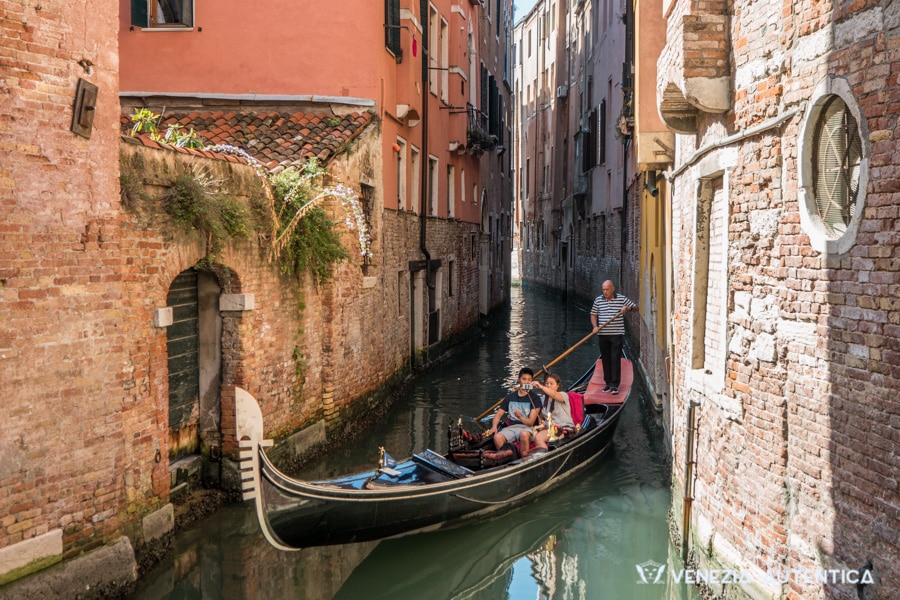The photograph captures a gondola navigating through a narrow canal in Venice, with vibrant color and detail. The gondola, black with a gentleman steering at the stern with a long oar, is adorned with a pink soft sheet. The gondolier, dressed in dark trousers and a horizontally striped black and white shirt, props himself at the back. Inside the gondola sits a young tourist couple, with the woman positioned slightly behind the man, who is almost in her lap. She is using her left hand to either point or take a photo. The couple is dressed casually in t-shirts and shorts.

The canal is flanked by buildings on both sides. The lower portions of these buildings are built from red brick, while the upper parts display a variety of pastel stuccos in shades from salmon pink to cream white. Some windows feature white frames, and terracotta shingles adorn rooftops. Several buildings even have greenery sprouting from their brick exteriors, along with visible drain pipes.

In the right-hand corner of the photograph, white text is partially obscured by the bright background, suggesting it may relate to "Venezuela," though it’s difficult to decipher. The buildings include circular windows and roof tiles, enhancing the scene’s picturesque quality. The sun casts light from the left, illuminating the canal and giving life to the enduring charm of Venice.